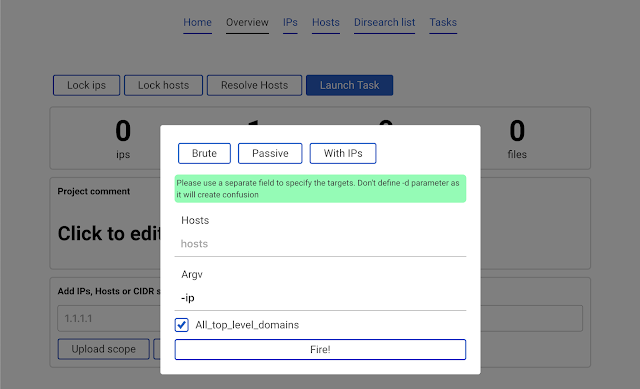In this image, we are looking at a computer screen displaying an application interface within a larger desktop screen. The main screen we see is bright white and acts as the focal point. At the top of this bright white interface, there are three options in a navigational toolbar. The first option, "BRUTE," is highlighted within a blue rectangle. Next to it are "PASSIVE" and "WITH IPS."

Below this toolbar, there is a green rectangle containing instructional text: "Please use a separate field to specify the targets. DON'T DEFINE /D parameter as it will create confusion." Following this text, there are several elements listed: "HOSTS" in all capital letters and "Hosts" with only the first letter capitalized. Beneath these, there's a label "ARGV" followed by "/IP."

Further down the page, a checkbox is ticked next to the label "All top-level domains." At the bottom of this white screen, there is a long rectangular button labeled "FIRE!" which appears to be clickable.

In the background, partially obscured by the bright white screen, we see a darker home screen interface with a menu on the left side. This menu includes options labeled "HOME," "OVERVIEW," "IPS," "HOSTS," "DEER SEARCH LIST," and "TASKS." Below these menu options, there are additional choices: "LOCK IPS," "LOCK HOSTS," "RESOLVE HOSTS," and a blue rectangular button labeled "LAUNCH TASKS." 

To the left of the main white interface, in bold letters, we can see the partially obscured text "CLICK TO EDIT," suggesting that some elements behind the white screen may be editable content. The bright white screen is overlapping much of the darker interface behind it, blocking out portions of the background information.